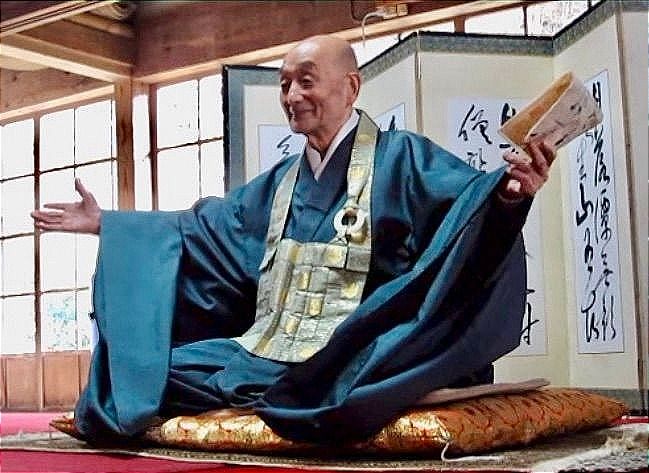In a serene, softly lit room suggestive of a traditional Japanese or Chinese setting, an elderly, bald man in a meditative pose sits cross-legged on a gold pillow adorned with red rings, situated atop a brown mat on a red floor. Dressed in long, flowing bluish robes with a grayish vest draped around his neck, he extends his arms out as if embracing the world, his left hand holding a folded parchment with visible ink bleeding through. His gaze is directed to his left. Behind him stands a freestanding Chinese partition adorned with papers inscribed with Asian script, partially obscuring large windows framed with light wooden panels. The scene radiates tranquility and profound contemplation, capturing a moment of serene introspection.